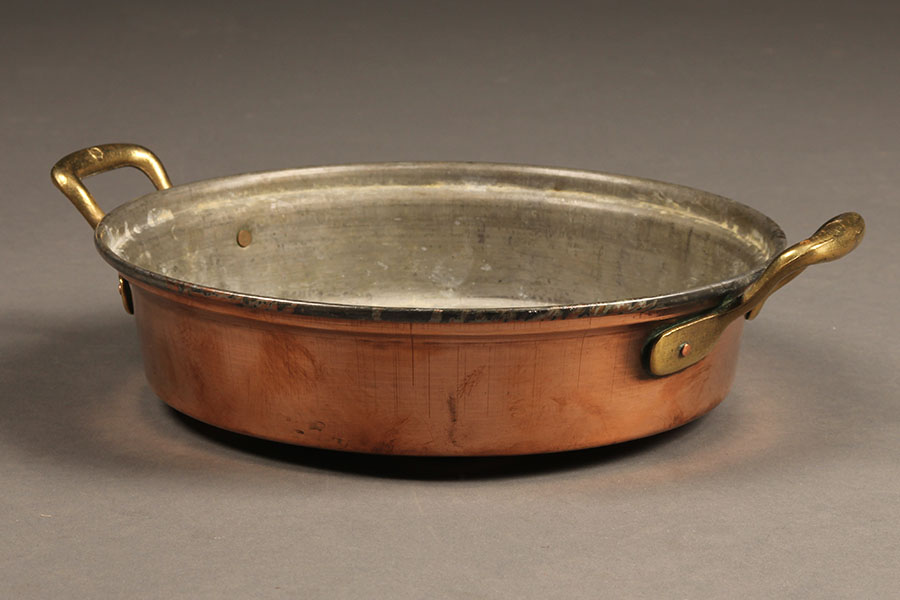This is a photograph of a copper pan, taken in landscape orientation. The pan sits on a gray surface, with its reflection faintly visible. The overall shape of the image is rectangular. The outer body of the pan is copper-colored with a thin metal frame circling the top edge. It features two ornate brass handles, one on each side, which are attached with golden screws. The interior of the pan is silver in color and appears empty, with some chalk-like residue along the sides and bottom. The lighting casts a subtle shadow beneath the pan, emphasizing its rounded shape akin to a shallow Dutch oven.